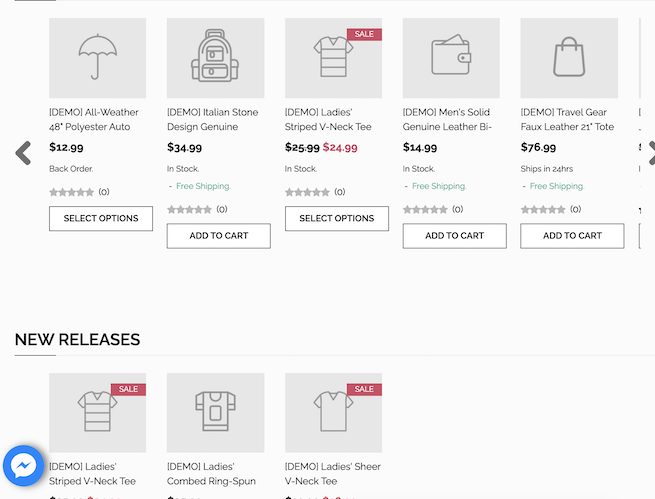This is a detailed screen capture of an ambiguous website displaying various retail products. At the top of the screen, there are five grayscale icons against a lighter gray background.

1. **Demo, All-Weather 48-inch Polyester Auto Umbrella**: Priced at $12.99 and currently on backorder. There's a "Select Options" button beneath the listing.

2. **Demo, Italian Stone Design Genuine Leather**: Priced at $34.99 and in stock at Descartes.

3. **Demo, Ladies Striped V-Neck Tee**: Marked as on sale with a banner indicating the original price of $25.99, now reduced to $24.99, and is in stock. There is also a "Select Options" button available.

4. **Demo, Men's Solid Genuine Leather Belt**: Partial description follows "by" and is cut off. Priced at $14.99, in stock at Descartes, and includes free shipping.

5. **Demo, Travel Gear Faux Leather 21-inch Tote**: Priced at $76.99 with a shipping time of 24 hours at Descartes.

At the bottom of the screen, three new releases are partially visible:

1. **Ladies Striped V-Neck Tee**: On sale.
2. **Ladies Combed Ring Spun Tee**: Details partially cut off.
3. **Ladies Sheer V-Neck Tee**: Details also partially cut off.

The image's context or the website it belongs to remains unclear.